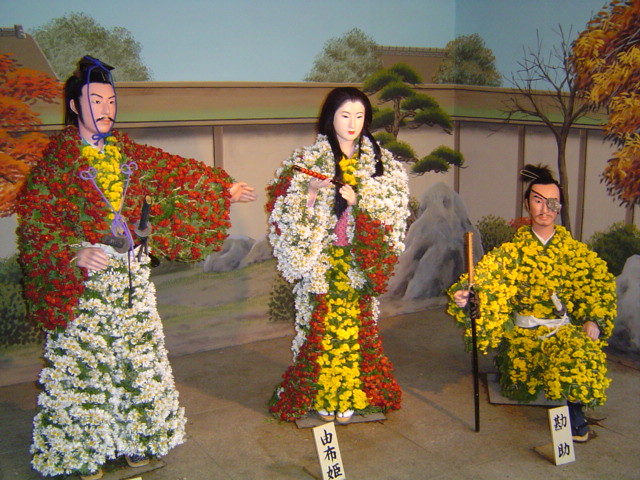The photograph captures an intricately detailed museum exhibit featuring three life-sized, wax-like statues of figures of apparent Asian descent, possibly Chinese. Each statue is dressed in elaborate attire made entirely of flowers, displayed against a realistically painted backdrop that depicts a serene garden with large rocks, trees, and a tan wall topped with brown. Two white signs with black Chinese text are positioned at the bottom center and right corner of the exhibit, possibly indicating the names or descriptions of the individuals.

On the left, a male figure stands with a black mustache and a blue ribbon tied around his head. His attire consists of a green and red floral coat with a yellow undershirt adorned with green flowers and a white and green floral skirt. He has a samurai sword attached to his waist, with one arm extended outward and the other close to his body.

The central figure, resembling a geisha, stands with a very pale face, red lips, and black hair cascading down her front. She wears a predominantly white costume interspersed with yellow flowers down the center and red and green flowers at the bottom. Her hands, holding a flute or cylindrical object, rest gently at her sides.

To the right, a kneeling male figure is dressed entirely in yellow flowers with green leaves, accented by a white belt around his waist. He wears an eye patch over his left eye and holds a sword with a brown handle and black blade. His entire costume complements the floral theme of the exhibit.

The background features a blue sky, green and brown trees, some with colorful blossoms, and grey rocks paving a serene, garden-like setting. The overall scene is a harmonious blend of historical representation, nature, and artistic floral costume design, making it a captivating exhibit within the museum.